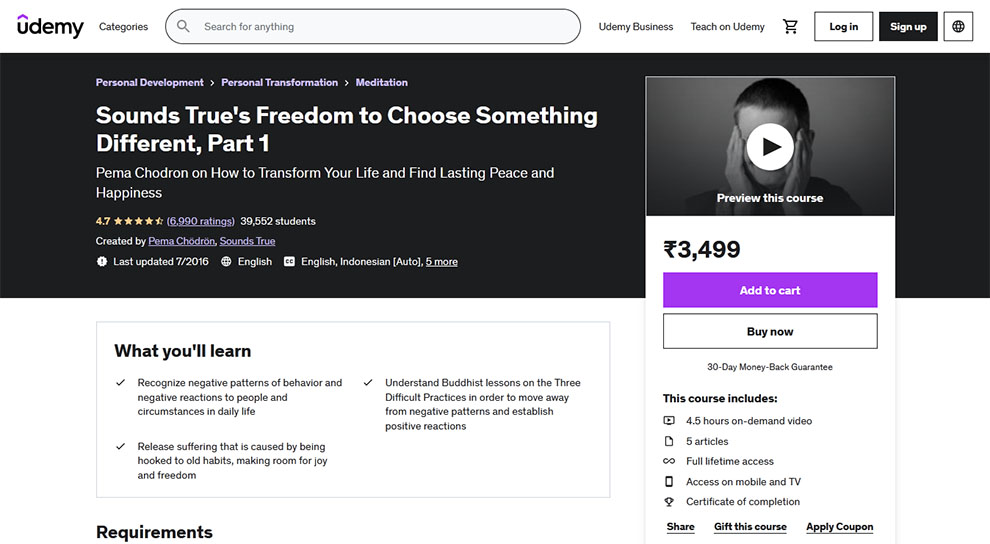**Caption:**

The top header features a black square with "Line Up" and a white square with "World." Beneath, there's a section for "Personal Development," "Personal Transformation," and "Meditation," emphasizing various themes such as sounds, trees, and freedom. The course, titled "Choose Something Different: Part One," is presented by Pema Chodron, aiming to transform your life and achieve lasting peace and happiness.

The course boasts a rating of 4.7 stars from 6,990 reviews and has 39,552 students. It was created in English, with subtitles available in English and Indonesian. The objectives of the course are to help you recognize negative behavioral patterns, release suffering from past habits, make room for joy and freedom, and understand Buddhist teachings on the three difficult practices to foster positive change.

Additional details include the course cost of $34.99, marked within a purple rectangle, and a "Buy Now" button with a 30-day money-back guarantee. The course package includes 4.5 hours of on-demand video content, 5 articles, full-time access, availability on mobile and TV, and a certificate of completion. Options to share, gift, or apply a discount coupon are also available.